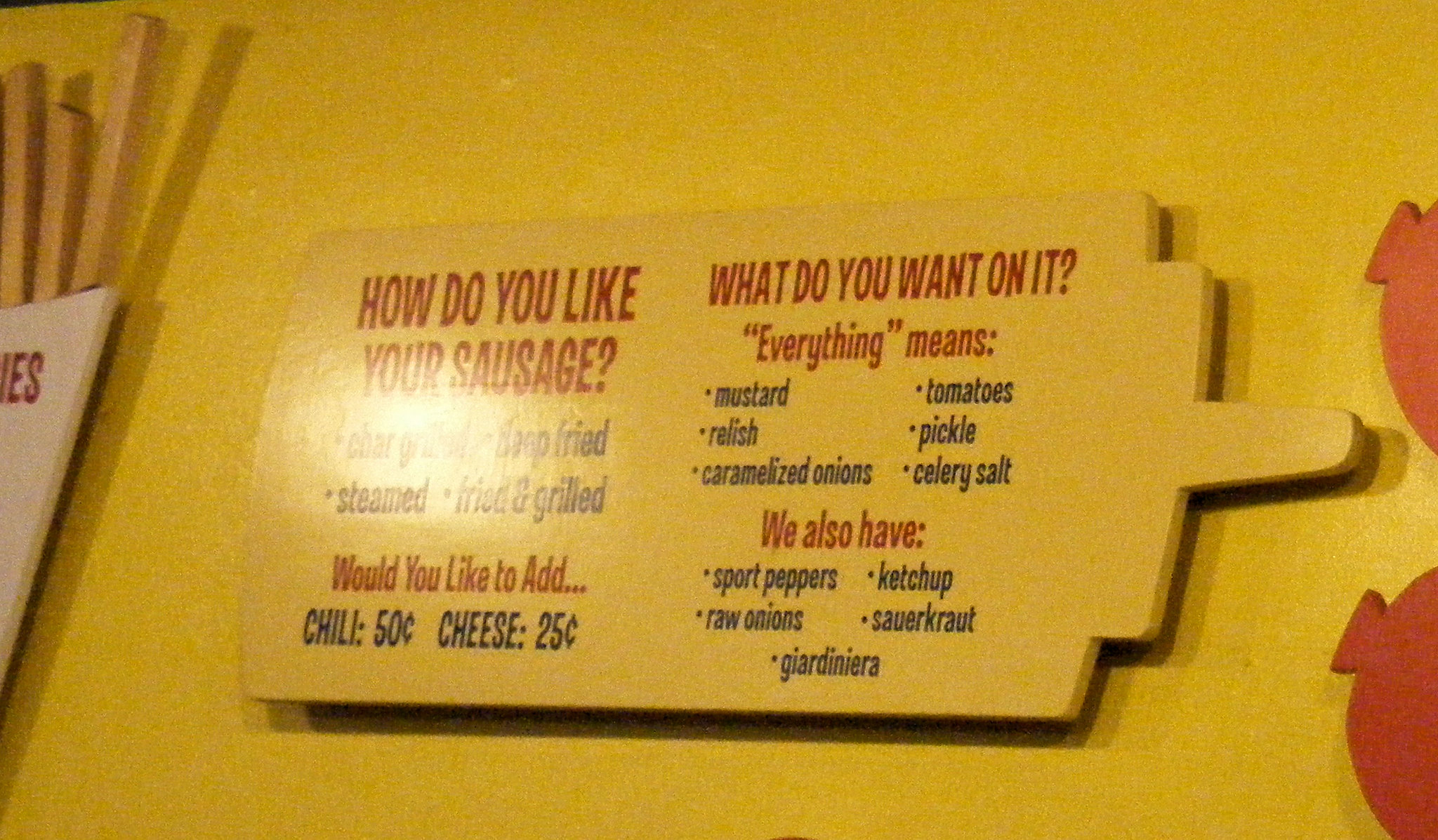The image depicts a vibrant yellow sign inside a restaurant, designed to resemble a flat rendering of a cylindrical condiment bottle, complete with a cap and pointed dispenser on the right side. The sign prominently asks, "How do you like your sausage?" Below this, although some text is obscured by a camera flash, phrases like "seasoned," "fried," and "grilled" are partly visible. Further down, the sign offers options for adding chili or cheese for an additional charge, specifically 50 cents for chili and 25 cents for cheese. 

Beneath this section, the sign inquires, "What do you want on it?" followed by a comprehensive list of condiments: mustard, relish, caramelized onions, tomatoes, pickle, celery salt, sport peppers, raw onions, ketchup, sauerkraut, and giardiniera. 

The wall behind the sign is painted a matching bright yellow. To the left of the main sign, there is another sign featuring french fries protruding from a white holder, though only the letters "e" and "s" are discernible. On the right side of the main sign, two unidentified red objects are visible, adding a splash of additional color to the composition.